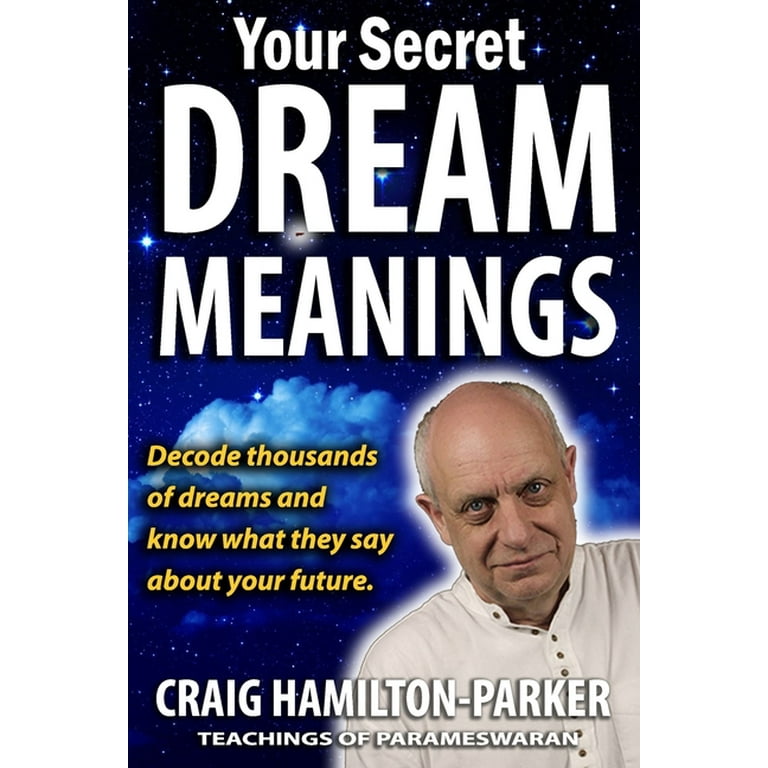The book cover is visually striking, featuring a blue background adorned with a night sky filled with stars and clouds, evoking a mystical and spiritual atmosphere. The title, "Your Secret Dream Meanings," is prominently displayed at the top in bold, white font, with the words "Dream Meanings" in all caps for emphasis. Below, in yellow text, it states, "Decode thousands of dreams and know what they say about your future," hinting at the book's promise to unlock the mysteries of dreams and their implications for one's destiny. 

Positioned at the bottom right corner of the cover is a smiling man, presumably the author, wearing a white shirt. His name, "Craig Hamilton Parker," is written below his image along with the phrase "Teachings of Parameswaran," adding an air of authority and expertise. The combination of deep blue and black hues, along with sparkling stars, contributes to the cover's enchanted and introspective feel, making it categorized under mystical or psychological genres with a spiritual undertone.